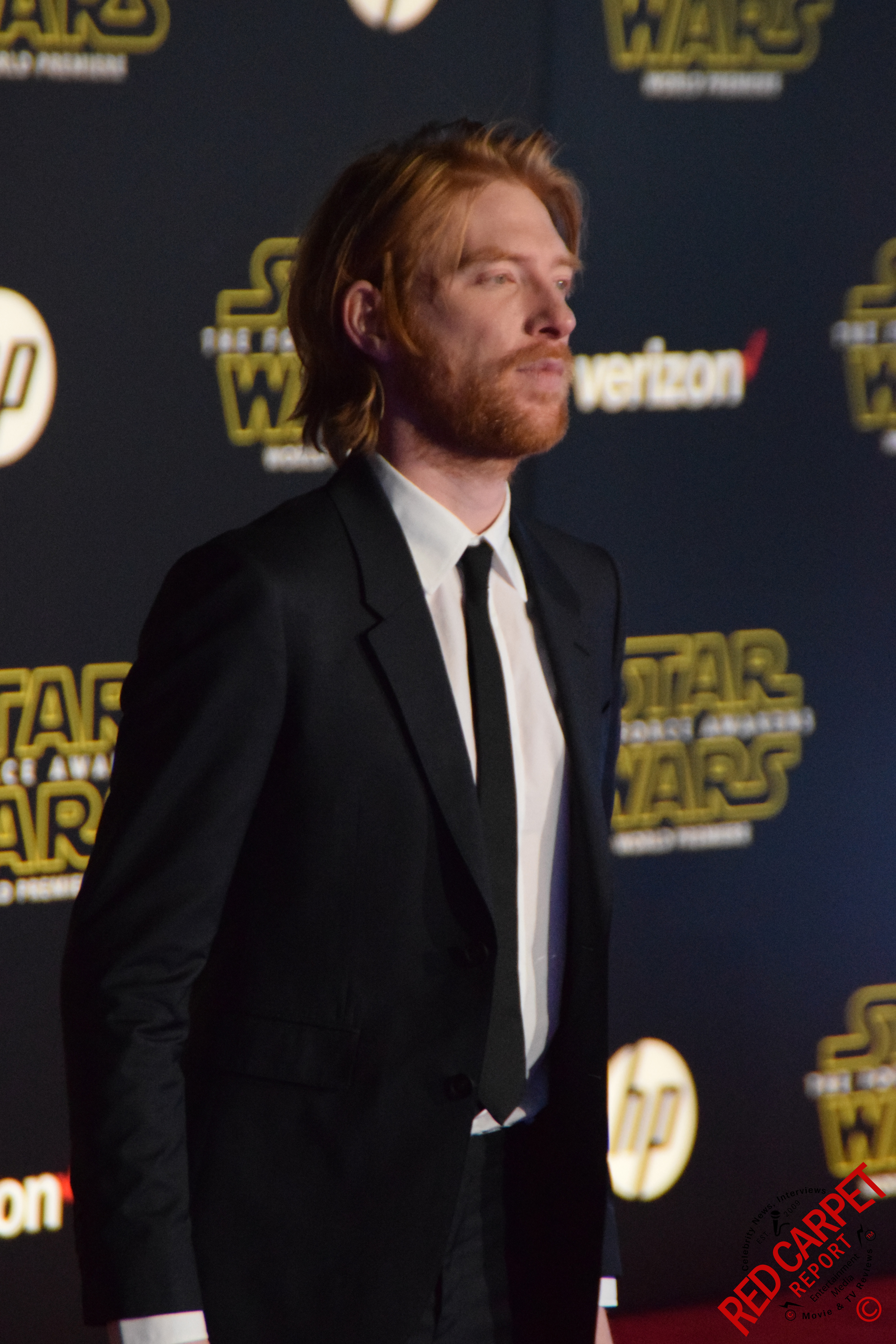This detailed image showcases a close-up photograph of a scruffy-looking man at a Star Wars premiere. The man features light brown, almost blonde hair that reaches his collar and a reddish-brown beard and mustache. He has freckles and is thin in appearance. His attire includes a black tuxedo, white collared dress shirt, black necktie, and black pants. In the background, a black wall prominently displays the logos of Star Wars, Verizon with a red checkmark, and HP. At the bottom right corner of the image, red text reads "Red Carpet Report" accompanied by a copyright symbol. The man is positioned looking towards the right side of the image with his back slightly turned to the left.